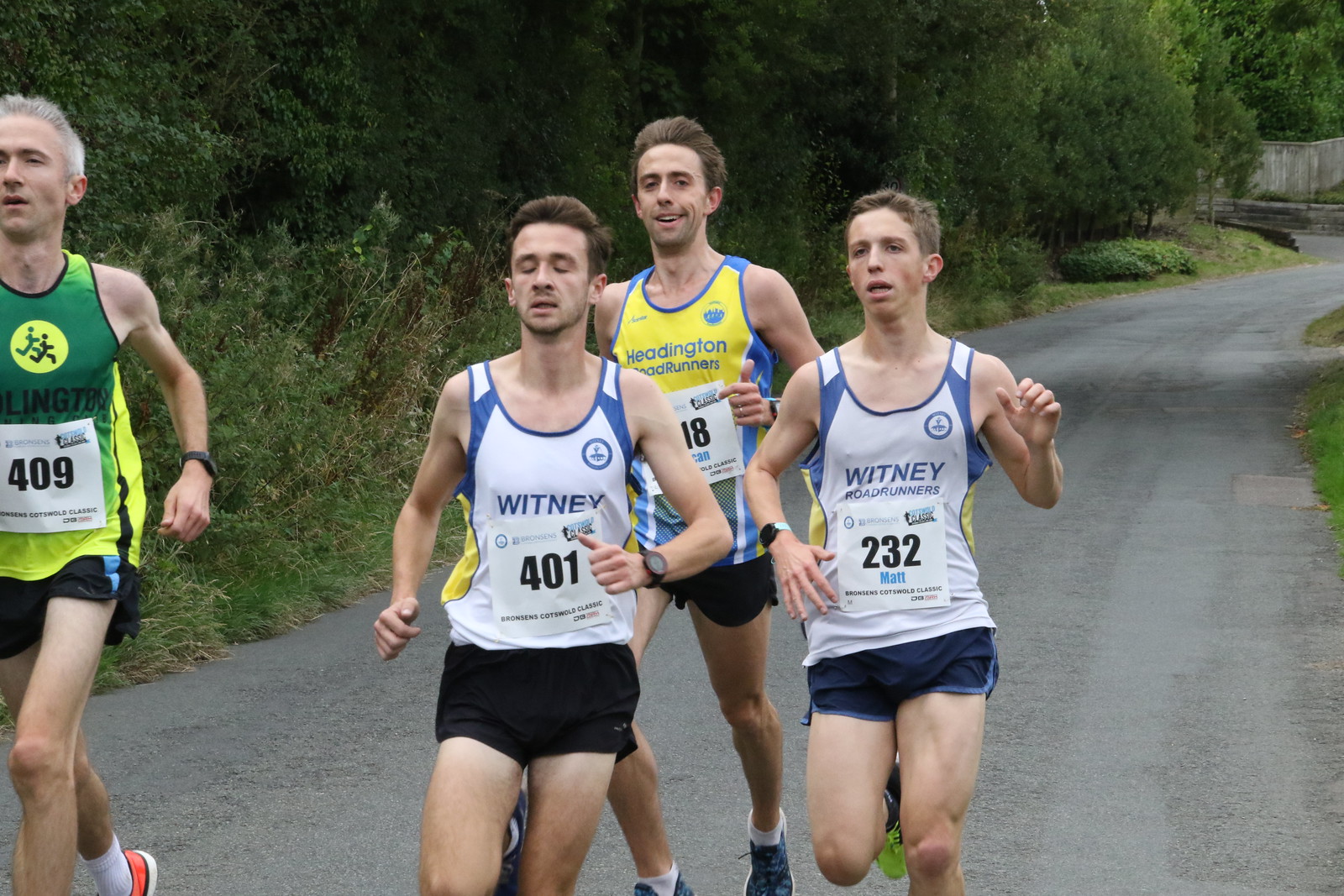The photograph captures a lively scene of four male runners participating in a race, evident by their race bibs displaying the numbers 409, 401, an obscured number ending in 8, and 232. They are running down a grey paved road lined with deciduous trees and green plants on the left and a small patch of grass on the right. Two men in the front are dressed in white tank tops with blue horizontal stripes on the shoulders, some yellow detailing, and the word "Whitney" emblazoned, paired with dark shorts. The runner on the right is wearing a yellow and blue tank top, with "Waddington Roadrunners" visible, while the man on the left-edge sports a green and yellow tank top. The three front runners have brown hair, and the fourth man, who looks directly at the camera and smiles, has grey hair. The image, set in broad daylight, showcases the men's focused expressions and dynamic movement, embodying the spirit of the race and the serene, lush countryside.